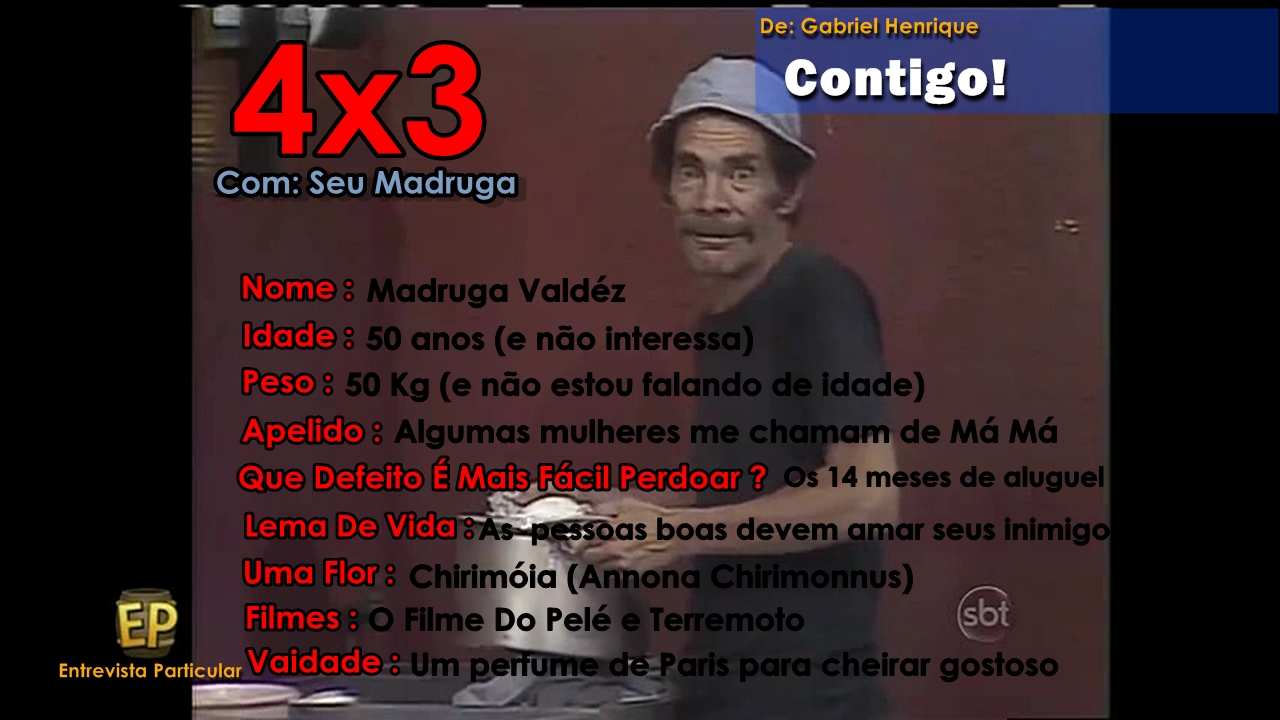The image is a screenshot likely from an older Portuguese-speaking television show or advertisement, showing a middle-aged man with dark hair, bushy eyebrows, and a big mustache. The man is wearing a gray bucket hat and a black shirt. He has wide, unsettling eyes and is holding a metal cooking pot. Superimposed on the image are numerous text elements: in the top right corner, it says "de Gabriel Henrique Contigo," and along the left side, starting from the top, it reads "4x3 com: su Madruga." Below that, additional statistics are given: "Nome: Madruga Valdez," "Idade: 50 anos," and "Peso: 50 kg." Other Portuguese phrases are also present, including "que de feito e mais facil perdor os 14 meses de aluguel" and "lema de vida: as pessoas boas devem amar seus inimigos." The entire presentation seems to be an interview or character profile, labeled "entrevista particular" on the left side.